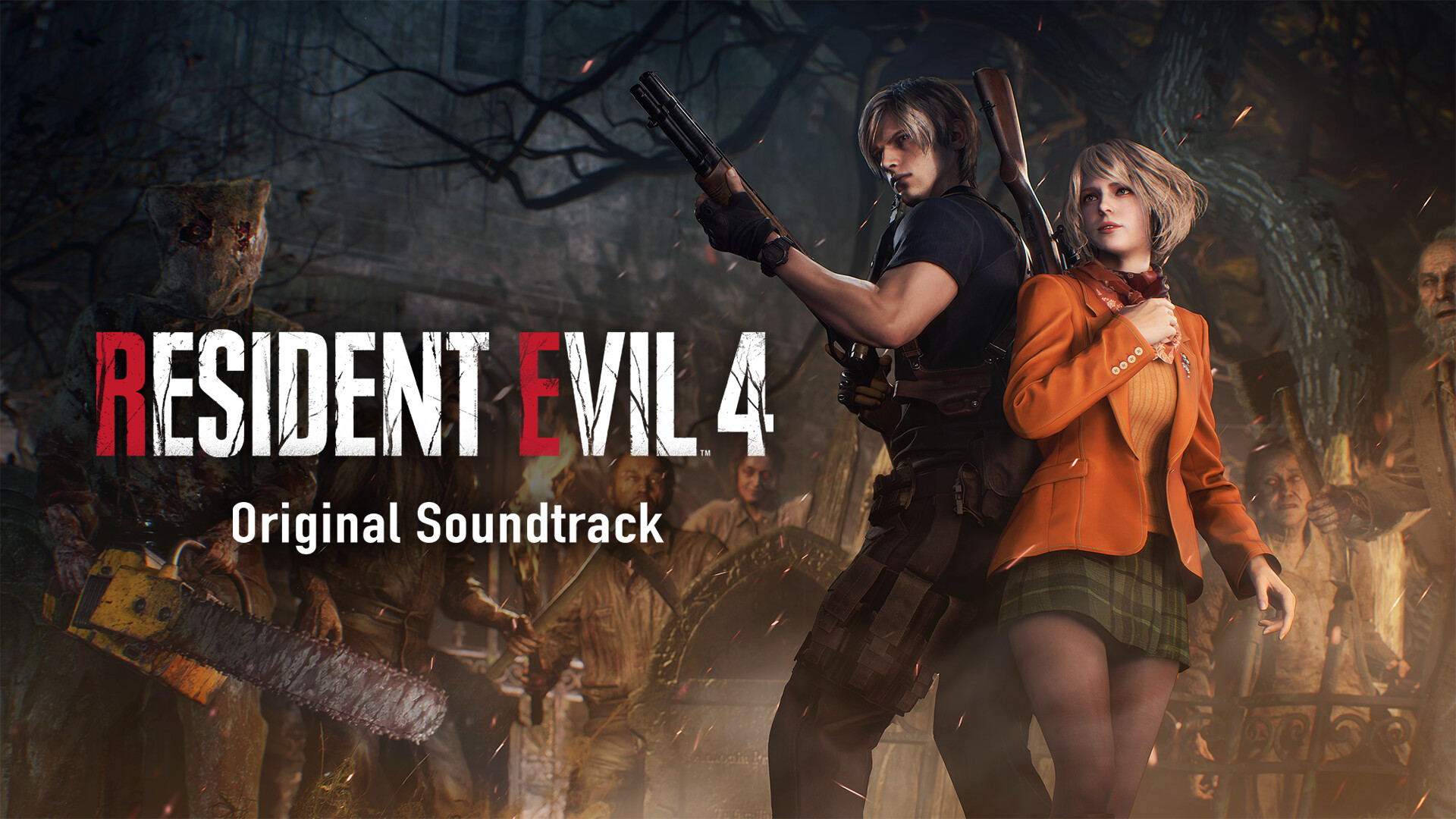The promotional banner for the Resident Evil 4 Original Soundtrack captivates with its dark and intense illustration, prominently featuring both heroic and menacing characters from the video game. The left side of the banner boldly displays the game's title, "Resident Evil 4," with the 'R' in 'Resident' and the 'E' in 'Evil' colored in red, while the rest of the letters and the number '4' are in white. Below the title, the text "Original Soundtrack" is also presented in white.

On the right side, the focus is on the two main characters, who stand back-to-back against a sinister backdrop of encroaching enemies. The male character is depicted in tan-colored cargo pants and a short-sleeved black shirt, wielding a pump-action shotgun with a break-action shotgun strapped to his back. The female character beside him has short blonde hair and is dressed in a short green plaid skirt, a blue coat, and an orange tank top, casting her gaze upwards. The scene is framed by a shadowy, ominous crowd, heightening the tension and danger embodied in the art.

Additionally, a figure on the left side, with a bag-like mask over their head and brandishing a menacing chainsaw, adds to the sense of dread. The dark background, teeming with a mob of hostile figures, reinforces the perilous atmosphere of the game, making this banner a dramatic and detailed representation of Resident Evil 4's eerie and action-packed experience.